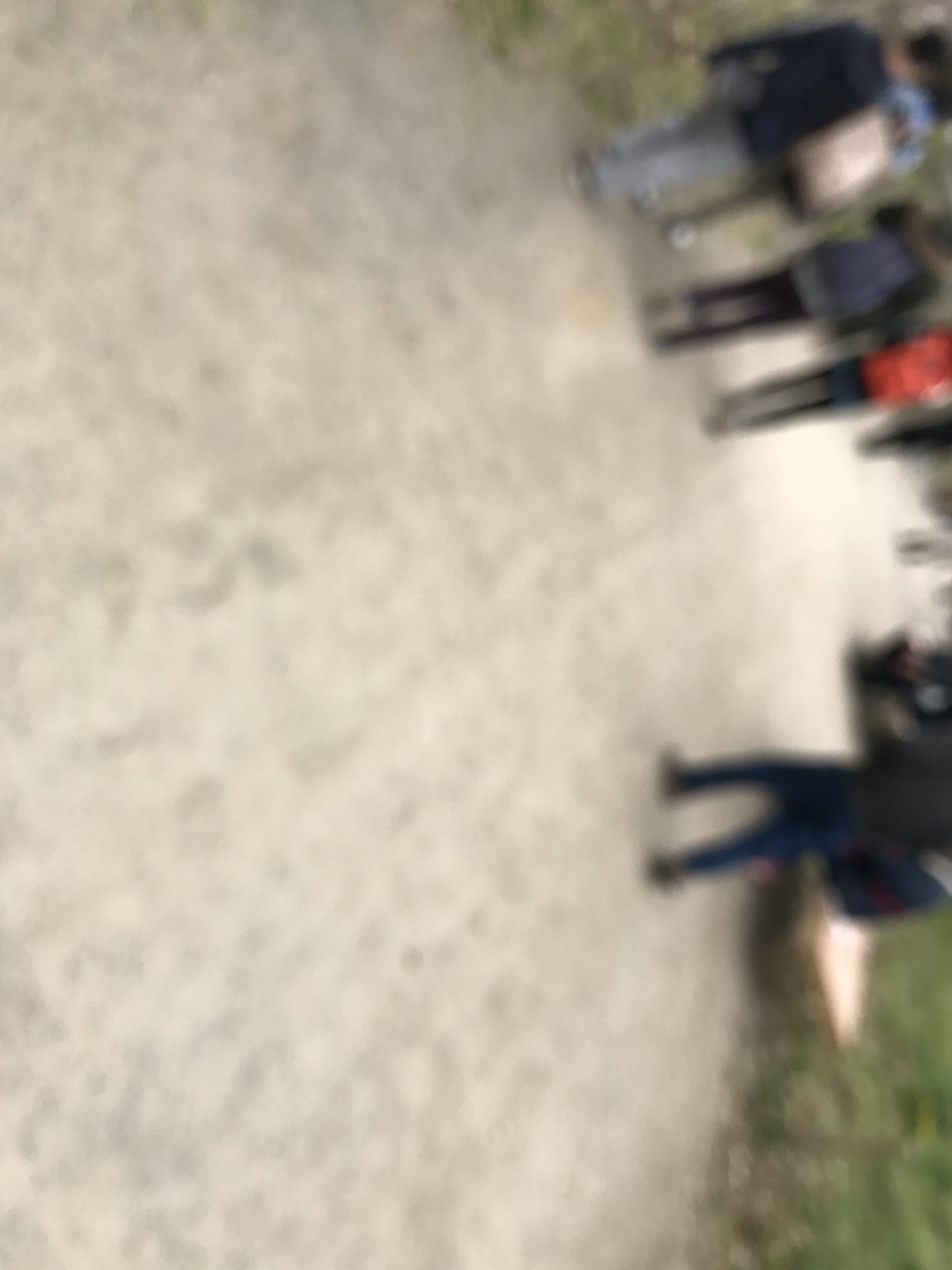This low-resolution, blurry image is oriented sideways, making it somewhat challenging to discern details. Nonetheless, several people are visible in the photograph. In the top right corner, there are faint outlines of a few individuals, though their features are indistinct due to the image's poor quality. Additionally, there is a person situated in the bottom right corner. Behind this individual, a green field of grass is noticeable, suggesting an outdoor setting. The people appear to be walking on a gray-colored path that runs through the scene. Despite the overall fuzziness and lack of clarity, these elements broadly characterize the image.